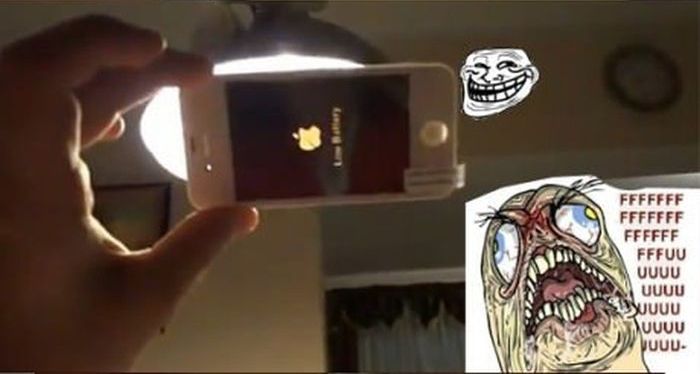The image is a dark, rectangular meme with a peculiar composition. On the left, a person's hand holds a white iPhone with a black screen, prominently displaying the white Apple logo. The phone is held in front of a bright light with a black lampshade, creating a stark contrast. To the right of the phone, there's a classic meme image of a troll face, a white face with an exaggerated grin penciled in with black outlines. In the bottom right corner, another cartoon face is visible. This face is tan, with white eyes accented by a bit of blue, an open mouth revealing white teeth and a pink tongue, and veins popping around its eyes, which glow red. Additionally, a series of letters are visible next to the cartoon face, with the first three rows containing the letter 'F' repeatedly and the bottom six rows filled with the letter 'U'. The overall focus of the meme is blurred and slightly compressed, adding to the chaotic and humorous aesthetic.